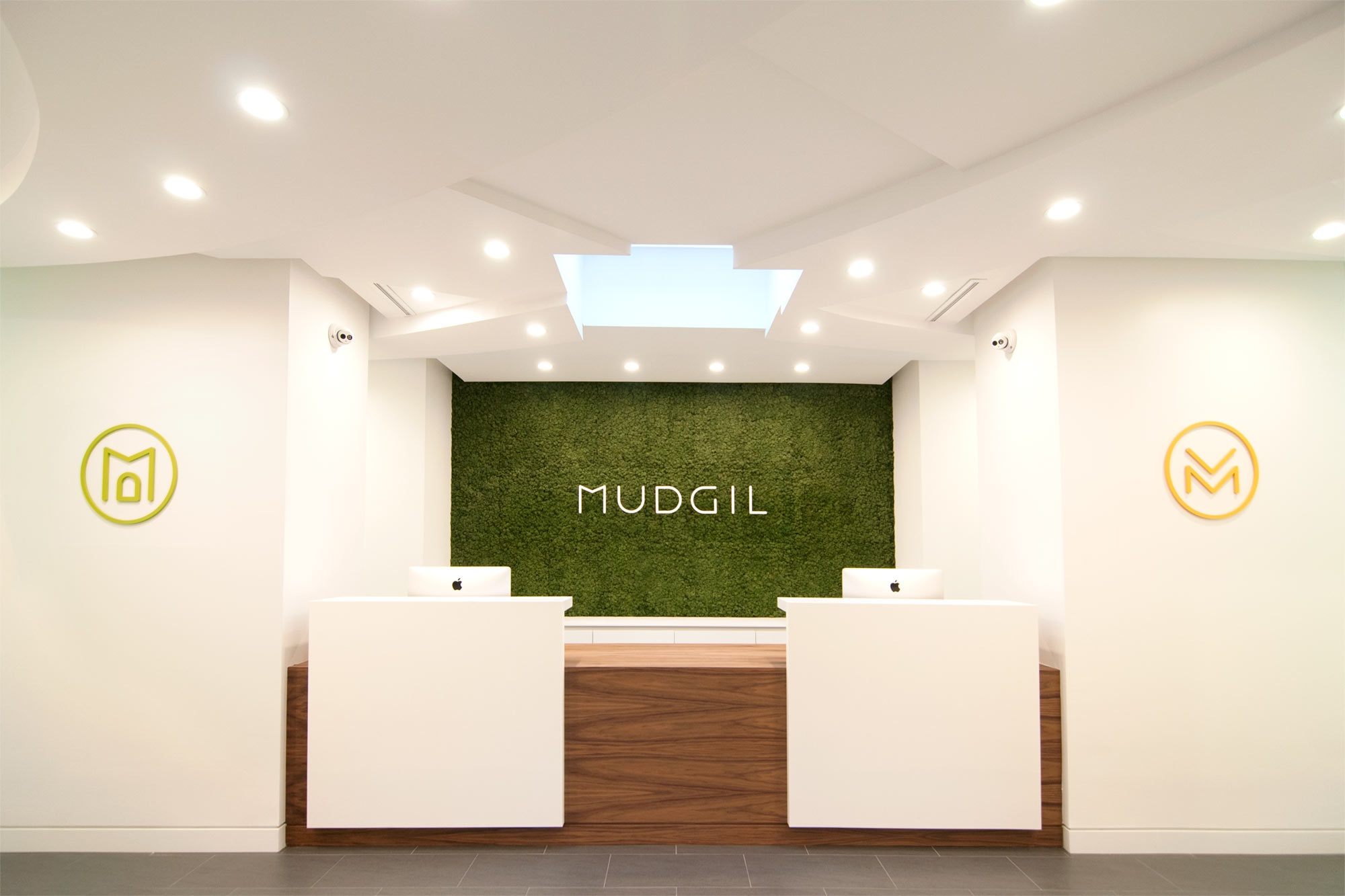The image depicts the reception area of a company or establishment named "Madgil." At the center of the image is a reception desk made from a brown, faux-wood material with two workstations, each equipped with a Mac computer on white stands. The desk features subtle black details that mimic the appearance of real wood. 

Behind the desk is a prominent green textured wall that gives off a natural, grassy appearance. Centered on this wall is the brand name "Madgil" displayed in a stylish font, possibly hanging. The contrasting white ceiling and surrounding walls brighten the space, highlighted by numerous pot lights that illuminate the area vividly. 

The flooring consists of matte gray tiles. Two logos adorn the space: one on the left wall, which appears as a circle containing an M that represents the entrance of a house with a doorway beneath it; and one on the right wall, also a circle with a stylized M intersected by an arrow pointing at the letter's middle section, rendered in a striking yellow.

No people are present in the image, which captures the sleek, modern design intended to welcome guests as they check in.